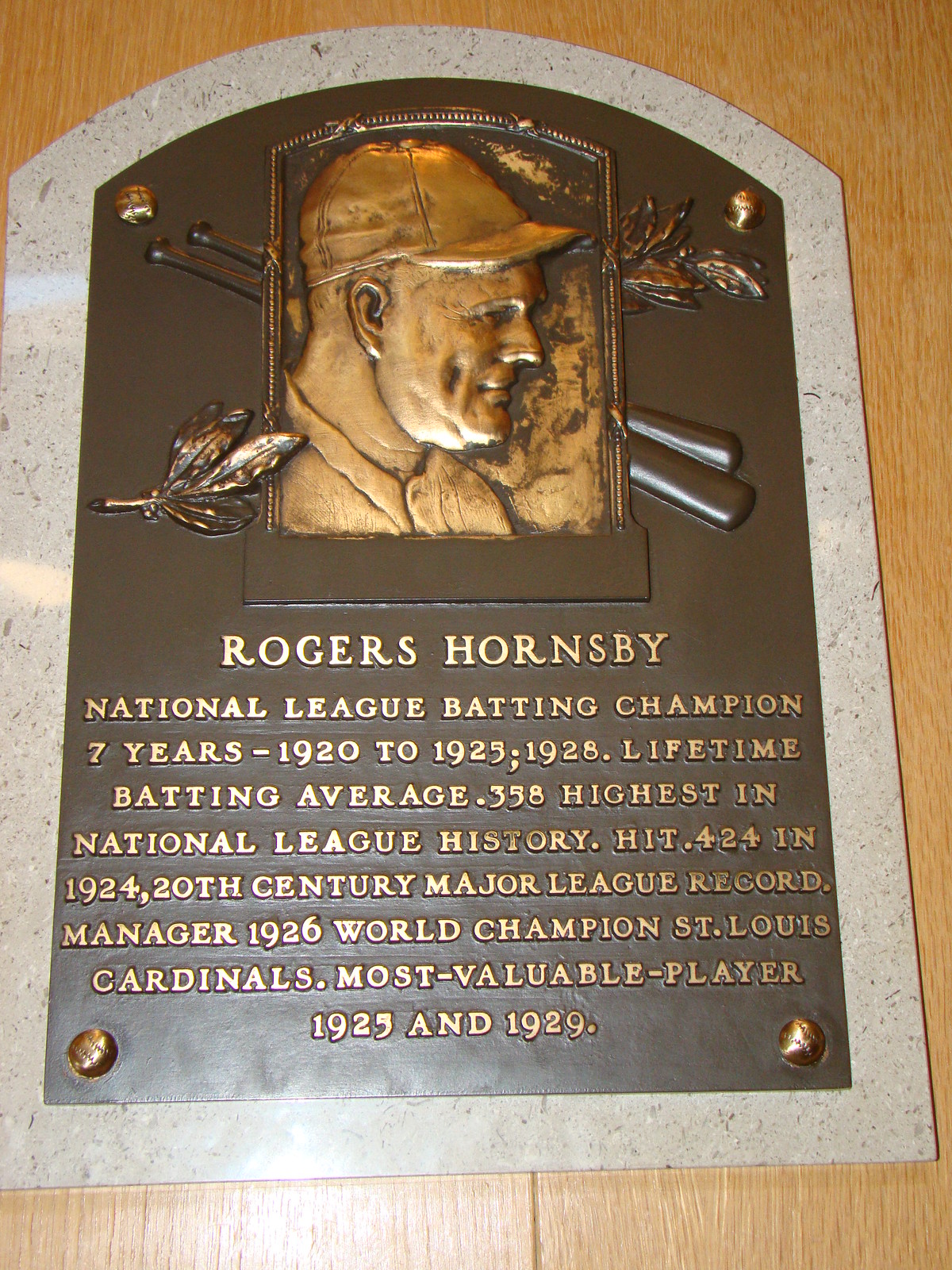The photograph captures a brass plaque dedicated to Rogers Hornsby, prominently mounted on a dark brown wooden wall. The plaque features a detailed brass relief portrait of Hornsby in profile, wearing a baseball cap, which extends just to the tops of his shoulders. Flanking the portrait are two baseball bats crossed behind him, intertwined with vines bearing leaves, adding an elegant decorative element to the piece. The inscription on the plaque reads in capital letters: "Rogers Hornsby, National League batting champion seven years, 1920 to 1925, and 1928. Lifetime batting average .358, highest in National League history. Hit .424 in 1924, a 20th-century major league record. Manager of the 1926 World Champion St. Louis Cardinals. Most valuable player in 1925 and 1929." The craftsmanship and contextual details of the plaque pay homage to Hornsby's exceptional contributions to baseball history.